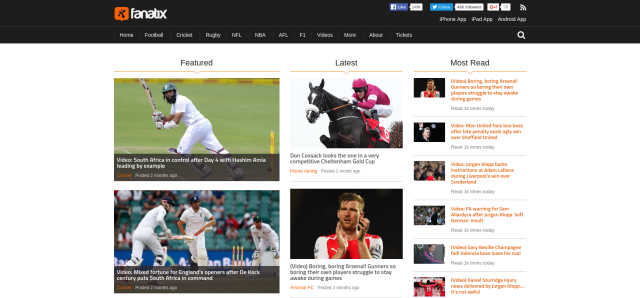The image displays a webpage from the sports website Fanatics. The webpage is divided into a "Featured" section and a "Latest" column, with multiple images and articles related to various sports events.

In the "Featured" section, the first picture showcases a cricket match. A man dressed in a white outfit, complete with a helmet strapped under his chin and knee pads, is holding a cricket bat with both hands. A yellow pole is visible to the right side of the image, set against a backdrop of green grassy fields. The scene also shows two additional players engaged in the game while another man, with hands on his knees, watches the action. The background includes fans seated in light blue chairs. The caption under the first cricket photo suggests that South Africa is in control after the fourth day, with player Haraham Amila setting an example. The second cricket image caption mentions Milford Fortune for England's spinners after a dialect century that challenges South Africa.

In the "Latest" column, the top image features a man riding a black horse, dressed in a red shirt, red helmet, and white pants. The number 5 is visible on the horse. Below this, another picture presents a man in an orange and white outfit.

Further down, there is a "Most Read" section listing six different articles, presumably detailing currently trending sports news and events.